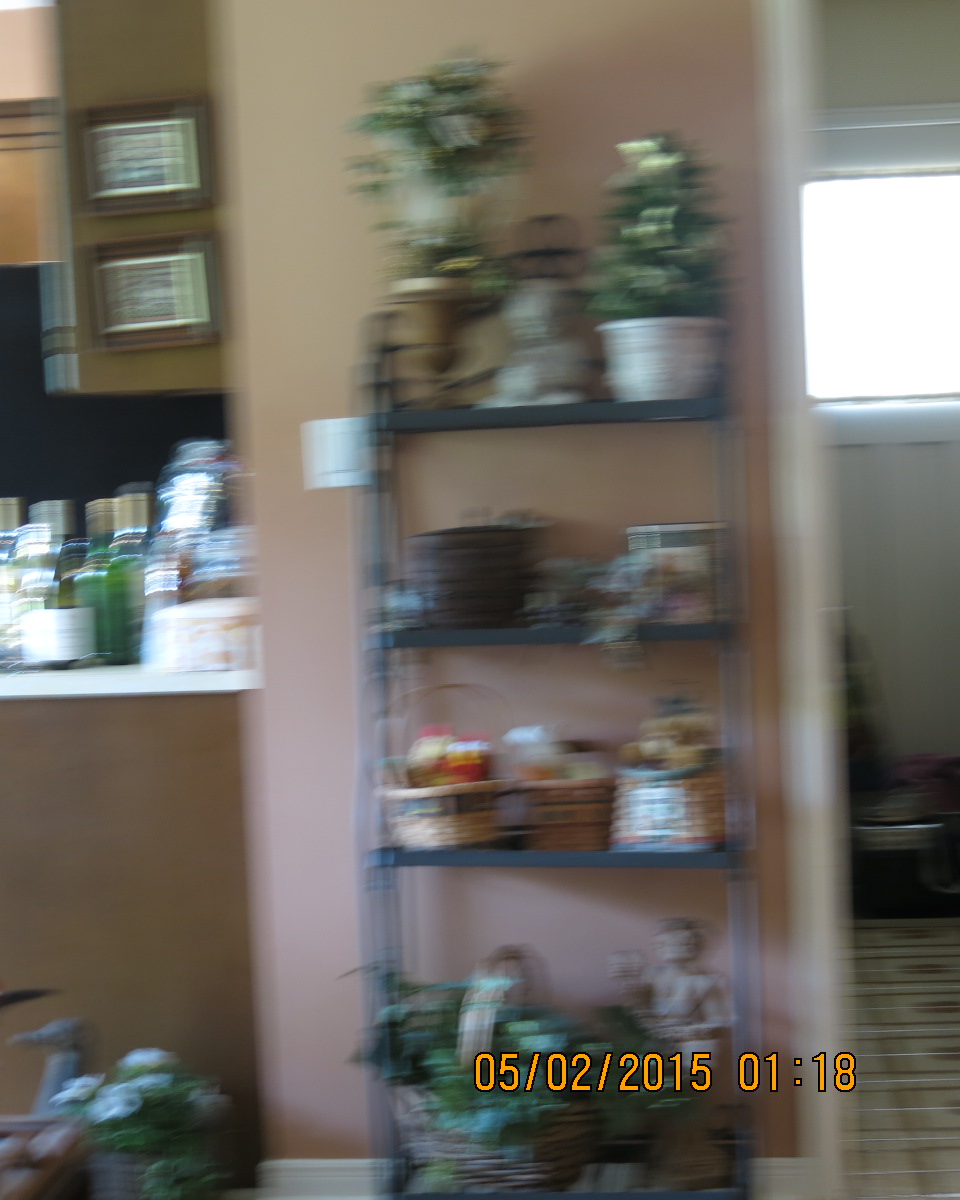This image is a blurry photograph taken inside someone's home, presented in a vertical rectangle shape. At the center, there is a small wall that appears to be beige or a very light shade of pink, featuring a gray metal four-tiered wire display shelf. On the top shelf, there are two potted plants and possibly other small pots. The second shelf holds a black pot along with other indiscernible items. The third shelf contains three baskets filled with various objects. On the bottom shelf, a basket with a green plant and a small statue can be seen. To the left of this wall, a white kitchen counter is visible with bottles on it, possibly alcohol. Above the counter, there are two framed pictures with white centers and brown outlines placed one above the other on a lighter extension of the wall. To the right, there seems to be a hallway leading to a door or window from which sunlight streams through. At the bottom right of the image, there’s a timestamp in orange text with a black outline that reads "05/02/2015 01:18."